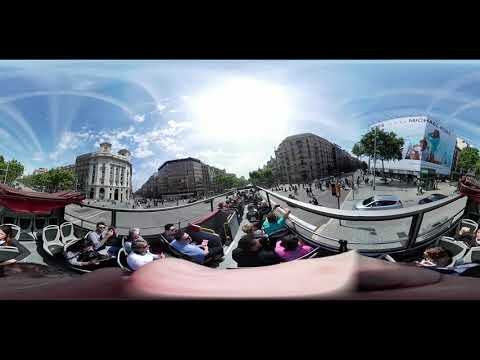The image is a color panorama photograph composed of two combined views in landscape orientation, capturing a vibrant city scene from the perspective of someone on a double-decker tour bus. At the top, the sky is a light blue with a bright white sun shining in the center, contributing to the overall realism of the image. In the middle distance stand several structures: on the left, a large light-colored building possibly indicative of a governmental function; to its right, a series of buildings including a brownish structure and further right, another large structure displaying a bent billboard.

The buildings on the right-hand side include one with an advertisement and another brownish building facing the street corner. The leftmost edge of the scene showcases a building with a distinctive red roof. Below these buildings, the bustling street includes a paved courtyard and curved fencing-like features. Amongst the street activity are parked cars and pedestrians. On the top level of the tour bus, men and women are seated in two-seater rows, looking out through curved, likely open-air windows, emphasizing the tourist atmosphere of the photograph. The blend of these perspectives through the panoramic filter encapsulates the lively urban environment they are exploring.